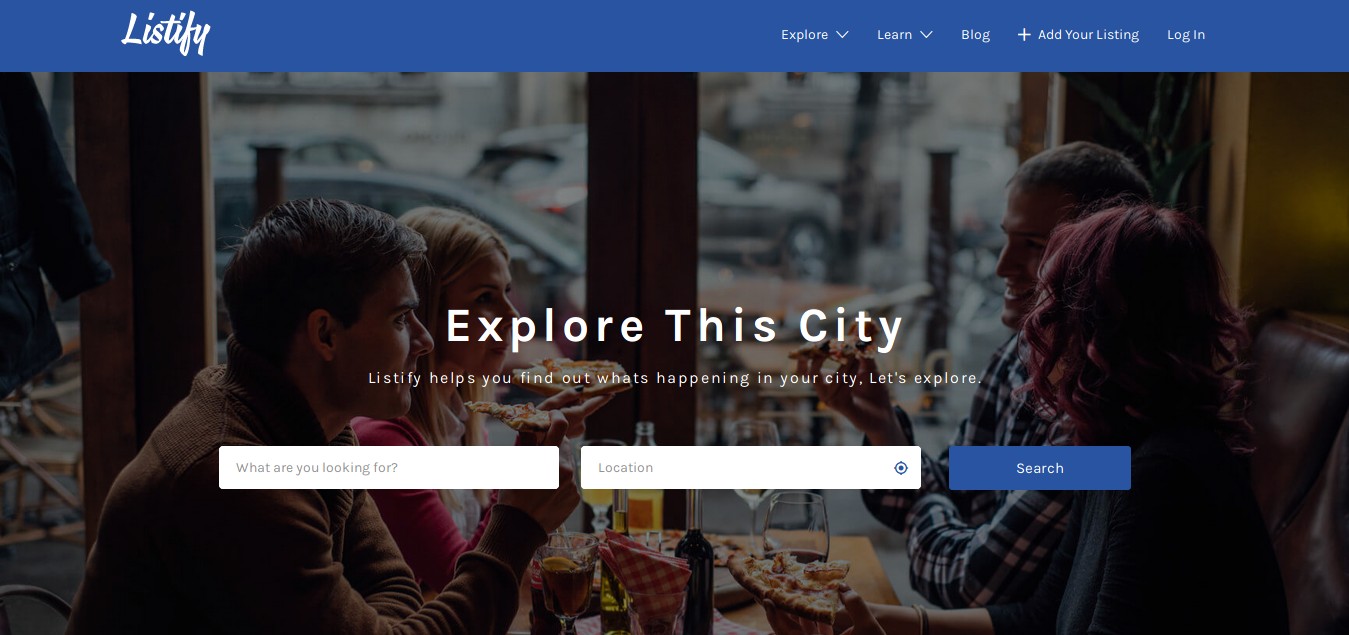This screenshot captures the homepage of a website named "Listify." The website's name, written in cursive, is located in the upper left-hand corner. A blue navigation bar spans the top of the page, featuring options such as "Explore," "Learn," "Blog," "Add Your Listing," and "Login" on the right side.

Below the navigation bar is an inviting image of four people—two men and two women—seated in a pizza restaurant, enjoying their time together. Superimposed over this image is the text "Explore This City," capturing the site's essence.

Underneath this headline, a tagline reads, "Listify helps you find out what's happening in your city. Let's explore!" Directly below the text, there is a white search bar with the prompt, "What are you looking for?" Additionally, a location field is available for users to enter their desired city or area. To the right of these fields is a blue search button, ready for users to click and begin their journey of discovery.